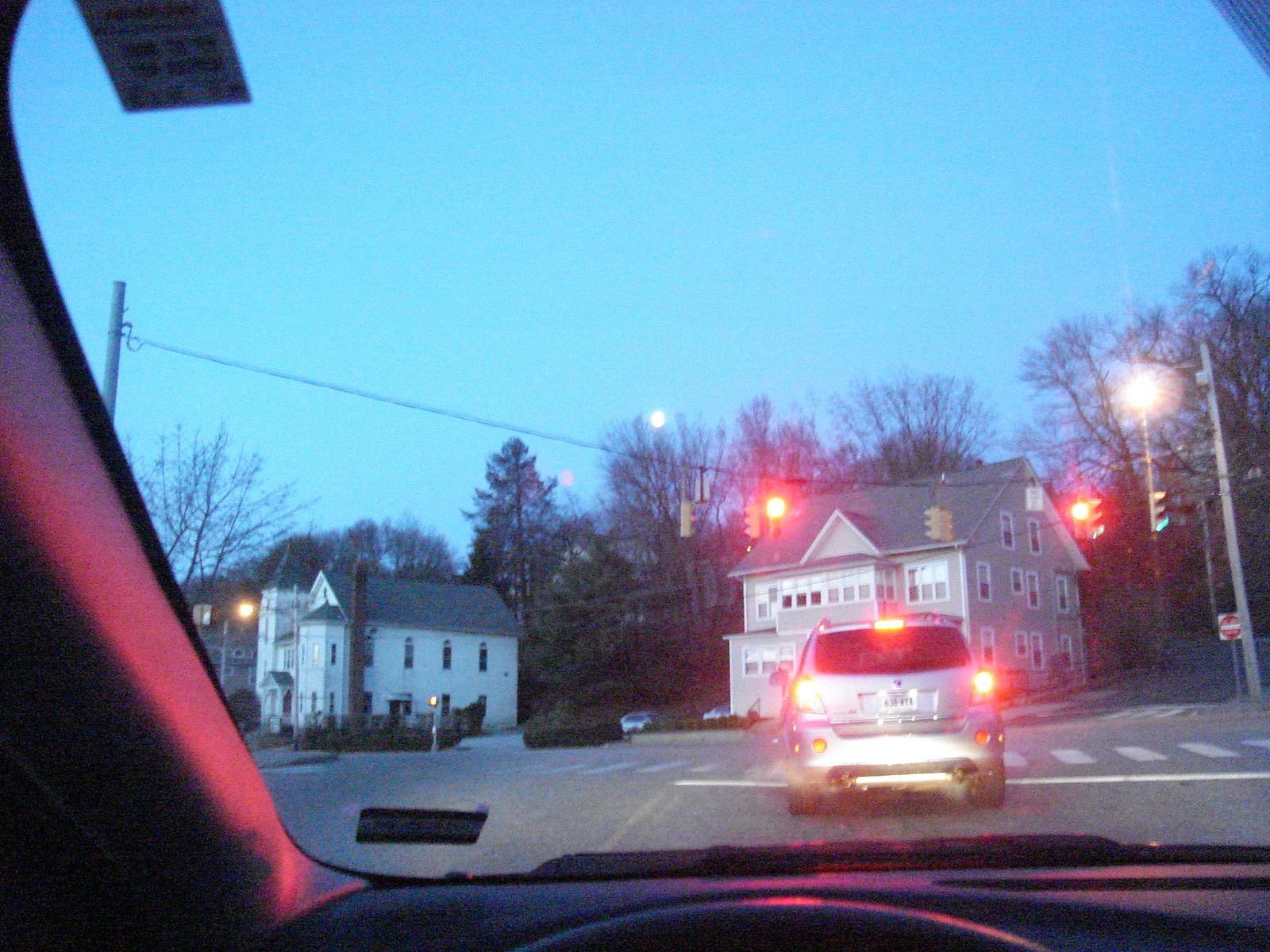The photograph, taken from inside a car, captures an urban scene at dusk. The tip of the vehicle's steering wheel is visible at the bottom edge of the image, suggesting the vantage point of the driver. In front, an SUV can be seen with its brake lights illuminated, indicating that it is stopped at a red traffic light. Adjacent to the red light, a green traffic light shines brightly, allowing cars from the perpendicular street to pass through the intersection. The immediate street is ending as it intersects with the cross street ahead, necessitating a turn for the driver. 

Further into the scene, several large houses or possibly townhouses line the street, their sizes imposing in the dim light. Streetlights have begun to cast their glow, illuminating the darkening streetscape. The scene takes place at sunset, contributing to the overall darkness, with only a hint of fading daylight visible in the sky.